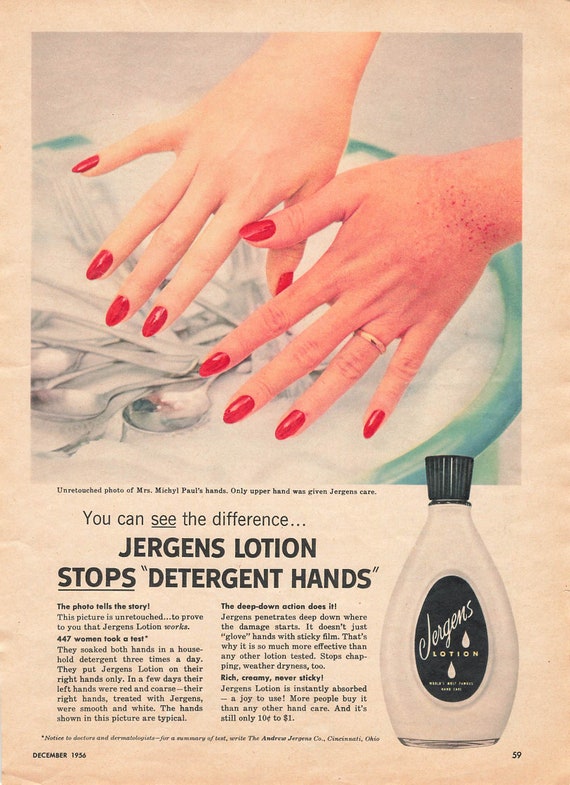This vintage magazine advertisement from December 1956 showcases the efficacy of Juergen's Lotion in combating "detergent hands." The ad features an unretouched photo of Mrs. Mitchell Paul's hands submerged in soap suds with silverware in a blue sink. Both hands are adorned with red nail polish, and the left hand bears a gold ring. The right hand, treated with Juergen's Lotion, appears smooth, white, and unblemished, contrasting the left hand, which is red, coarse, and wrinkled. The ad boasts the results from a test involving 447 women who soaked their hands in household detergent three times daily, revealing that only the right hands treated with Juergen's Lotion remained smooth and white. At the bottom, the text elaborates on Juergen's deep-penetrative action, claiming it stops chapping and weather dryness better than other lotions. The advertisement is visually complemented with an image of the Juergen's Lotion bottle, featuring a black top and label. It highlights the product's affordability, priced between ten cents and one dollar, and concludes with a notice to doctors and dermatologists for a test summary, provided by the Andrew Juergen's Co., Cincinnati, Ohio.